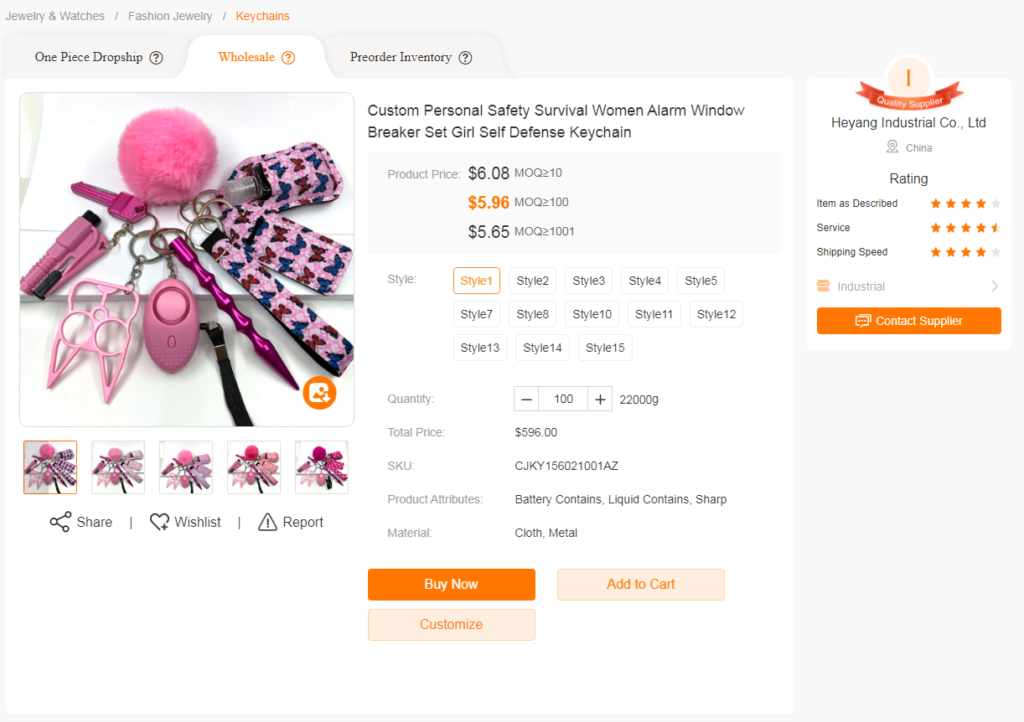This image depicts an online store webpage for a keychain product under the category path: Jewelry & Watches > Fashion Jewelry > Keychains. The specific breadcrumb "Keychains" is highlighted in orange. At the bottom of the page, the text reads "One-piece dropship wholesale pre-order inventory," with "wholesale" emphasized in orange.

The main product showcased is a customizable self-defense keychain set tailored for women, priced at $6.08, with discounts listed below to $5.96 and ultimately $5.65. This pink keychain set includes features like a personal alarm, window breaker, and other survival tools. The selected style on display is "Style 1" out of 15 available options. The page notes that the total price for a quantity of 100 units is $596. The product attributes include battery content, liquid content, and materials such as cloth and metal. 

The interface includes three interaction buttons at the bottom: "Buy Now" highlighted in orange, "Add to Cart" in a lighter shade of orange, and "Customize." In the top right corner, the supplier is indicated as Heiang Industrial Co., LTD from China, featuring ratings — 4 stars for item description, 4.5 stars for service, and 4 stars for shipping speed, all in orange. An orange button labeled "Contact Supplier" is also present.